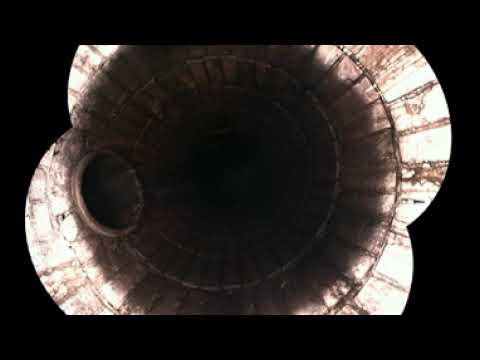The image is predominantly black, except for a central structure that draws the eye. At the center, there are four concentric circles that create a shape reminiscent of a four-leaf clover or a flower with four petals. These "petals" are white and exhibit pinkish-red, rust-like wear patterns radiating outward. The central area of this shape is darker, suggesting depth or a hole, with an inner circle that is difficult to discern.

Surrounding these concentric circles and petals are light brown stains, resembling worn-out concrete, that add texture to the form. The entirety of this intriguing, possibly industrial or spacecraft-related structure is set against a completely black background, making the details of the central image stark and prominent.